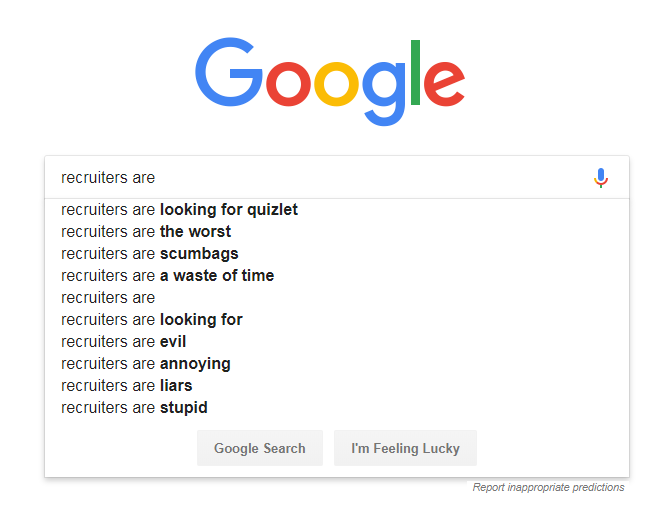The image depicts a screenshot of a Google search page. At the top, the colorful Google logo is prominently displayed, with the letters G, O, O, G, L, and E respectively colored in blue, red, yellow, blue, green, and red. Below the logo, a search bar shows the partially typed query, "recruiters are." To the right of the search bar, a multicolored microphone icon—blue, yellow, red, and green—indicates the voice search option.

The dropdown suggestions under the search bar include phrases such as "recruiters are looking for Quizlet," "recruiters are the worst," "recruiters are scumbags," "recruiters are a waste of time," and further autocomplete suggestions like "recruiters are blank," "recruiters are looking for," "recruiters are evil," "recruiters are annoying," "recruiters are liars," and "recruiters are stupid." 

At the bottom of the search interface, there are two gray buttons: one labeled "Google Search" and the other "I'm Feeling Lucky."